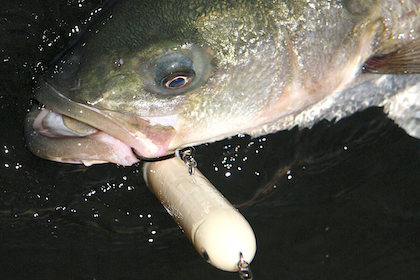In this close-up photograph, the head of a recently caught fish emerges from the water, still partially submerged and creating gentle ripples around it. The fish's dark green top and light gray sides lead to its partially open mouth, where a black hook is visibly lodged in its cheek. Attached to the hook is a beige, pill-shaped lure connected by a small metal chain, indicating the fish's capture. The fish's prominent eyes, large with black pupils and a golden yellow rim, gaze outward. The image details the fish's upper body, showing hints of its gills and the small fin on its left side against a backdrop of dark, rippling water, capturing the tense moment before the fish is either reeled in or released.